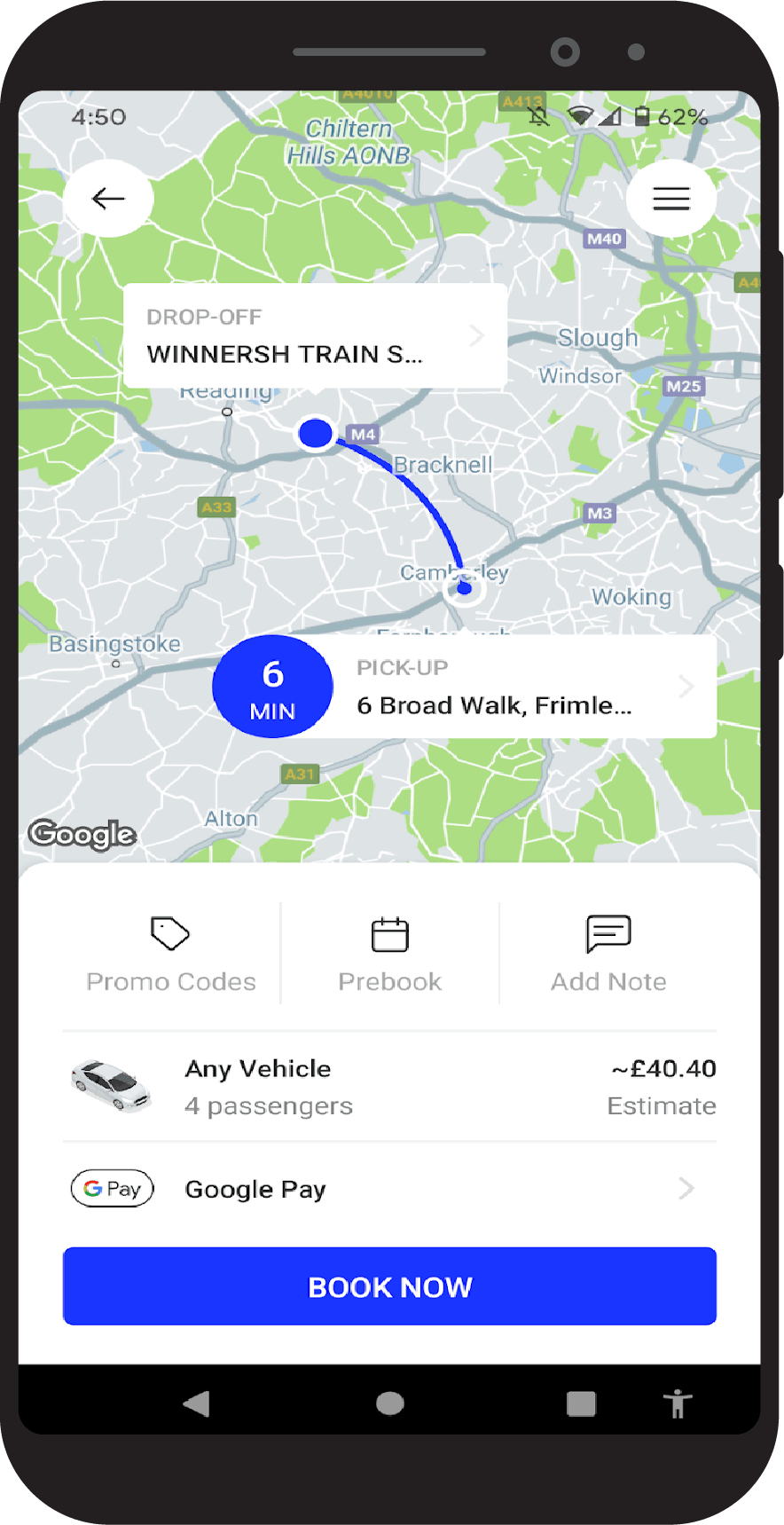A high-resolution image displays a smartphone screen with Google Maps open. The timestamp on the screen reads 4:50, and icons for Wi-Fi, notifications (which are turned off), and battery life (at 62%) are visible at the top. On the left side, a black arrow within a white circle points to the left, while on the right side, a hammer icon in a white circle is shown. 

The map indicates a route from the start location marked "Pick Up" at "6 Broad Walk, Fremantle" with an estimated travel time of six minutes. The destination is labeled "Drop-Off" at "Winner's Train Station," with further detail obscured by an ellipsis. 

Beneath the map, there are options to enter a promo code, pre-book the ride, or add a note. A faint gray line separates these options from an image of an automobile, which indicates the choice for "Any Vehicle" suitable for four passengers. The fare estimate is 40.40 Euros. 

Below the fare estimate, the screen highlights that payment can be made via Google Pay, whose logo is also present. A prominent blue "BOOK NOW" button invites the user to confirm the booking. 

At the very bottom, the smartphone's navigation bar is displayed with a left-facing light gray arrow, a home button, a stop button, and a user icon.